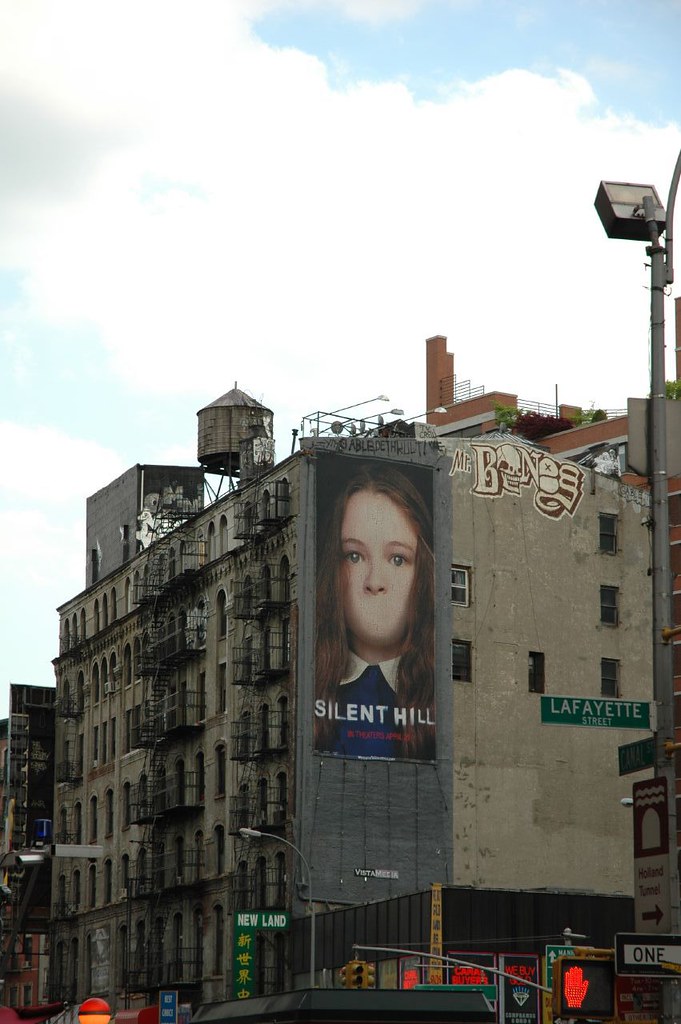The outdoor image features a large, aged building with a grayish-brown, somewhat dirty facade, spotted with graffiti including the word "bones" in brown. The mid-ground is dominated by this structure, which spans at least six stories, with rows of windows and several black balconies extending from its sides. On the roof lies a small water tower along with some long chimney pieces and fencing.

The ground level hosts a variety of stores, one prominently displaying the word "Newland" in white, capital letters against a green background. A traffic sign near the building shows a white pedestrian symbol, while directional signs indicate "Holland Tunnel" in brown, "Canal Street," and "Lafayette Street" in white capitals on green backgrounds.

Dominating one side of the building is a large, striking movie poster for "Silent Hill," featuring a young girl with long brown hair in a blue dress with a white Peter Pan collar. Her mouth is eerily missing, replaced by skin, and "Silent Hill" is written in bold, white letters below her image. The vibrant blue sky with puffy white clouds adds a contrasting backdrop to the gritty urban setting, capturing a surreal blend of everyday city life and unsettling cinematic advertisement.